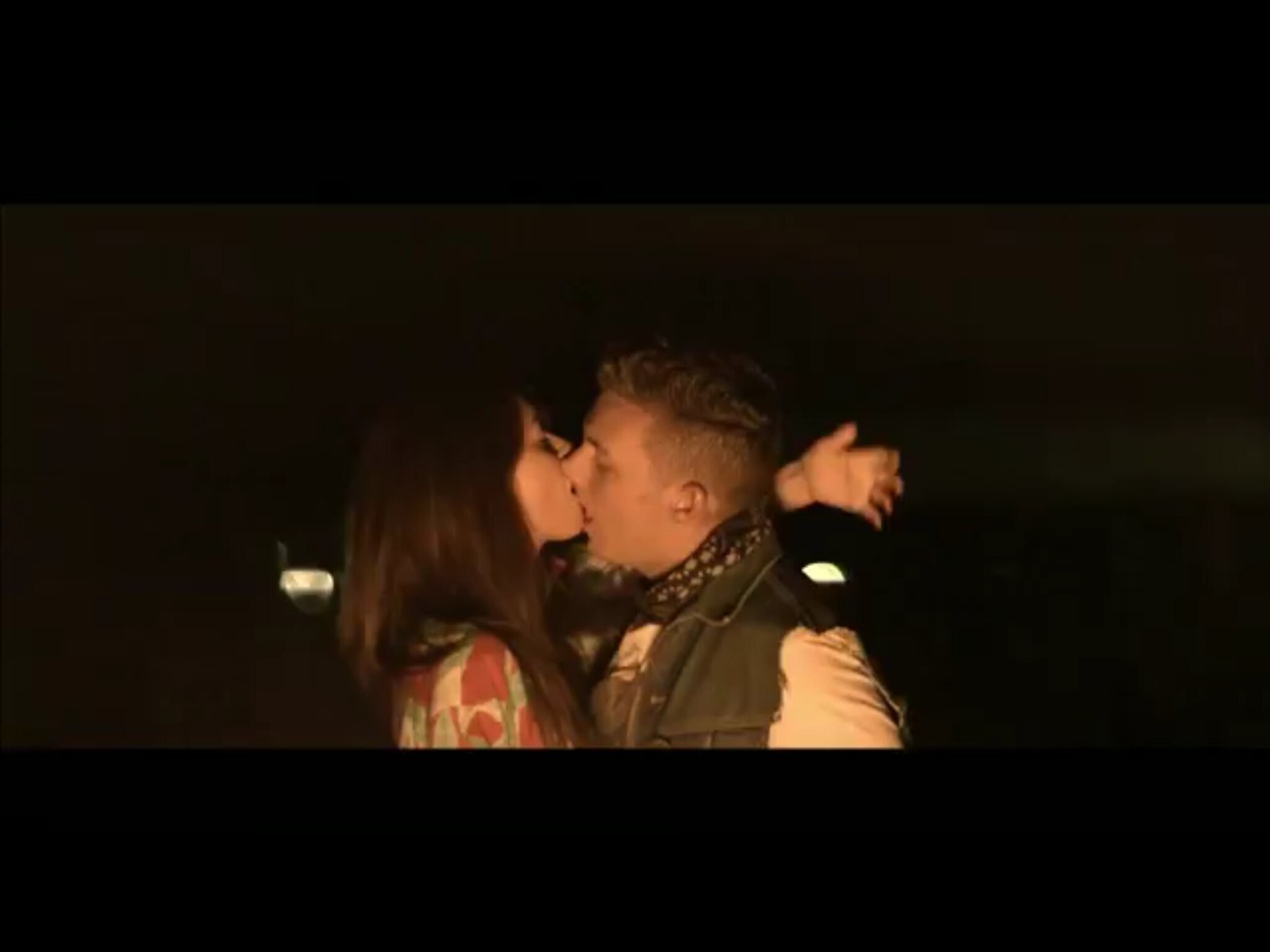This close-up photograph captures the intimate moment of a young couple kissing against a pitch-black background, suggesting it might be a frame from a movie or a nighttime outdoor setting. The woman on the left has long, silky brown hair cascading past her shoulders, and she is wearing a multicolored dress with a pattern of irregular red, green, and beige squares. Her eyes are closed and her mouth is slightly open, aligned a bit higher than the man's. Her left hand is reaching around to caress the back of his neck. The man on the right has short brown hair, buzzed around the ears and back with a spiked top. He is dressed in a white shirt layered under a dark green cut-off jacket and accessorized with a black and gray spotted scarf. Their profiles are prominently featured, set against the impenetrable darkness save for dimly illuminated car headlights in the background. The composition is framed by black bars at the top and bottom, adding to the cinematic feel of the image.